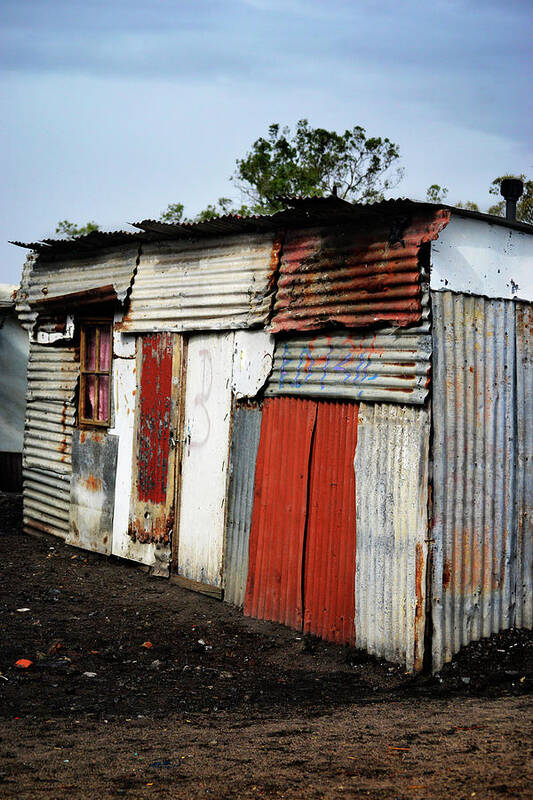The image depicts a small, roughly assembled structure that resembles a shed or an improvised home. The building is constructed from a patchwork of corrugated metal sheets in various colors, including reds, whites, grays, and blues, some of which are rusted or painted, with a few pieces covered in graffiti. The metal sheets are haphazardly arranged, giving the building a rustic, dilapidated appearance. Its roof is also composed of these corrugated metal panels, and a pipe extends from it, suggesting the possibility of heating inside.

A plain, weathered wooden door painted in white stands at the entrance, and to its left is a window adorned with a pink curtain. Surrounding the building is a barren expanse of gray and black dirt, devoid of grass, gravel, or pavement. The background features a clear, blue sky with no clouds in sight, and the top of a green foliage tree can be seen peeking into the frame. The overall scene suggests a resourcefully constructed dwelling, potentially indicative of low-income housing or a structure from an area where such homes are commonly built.